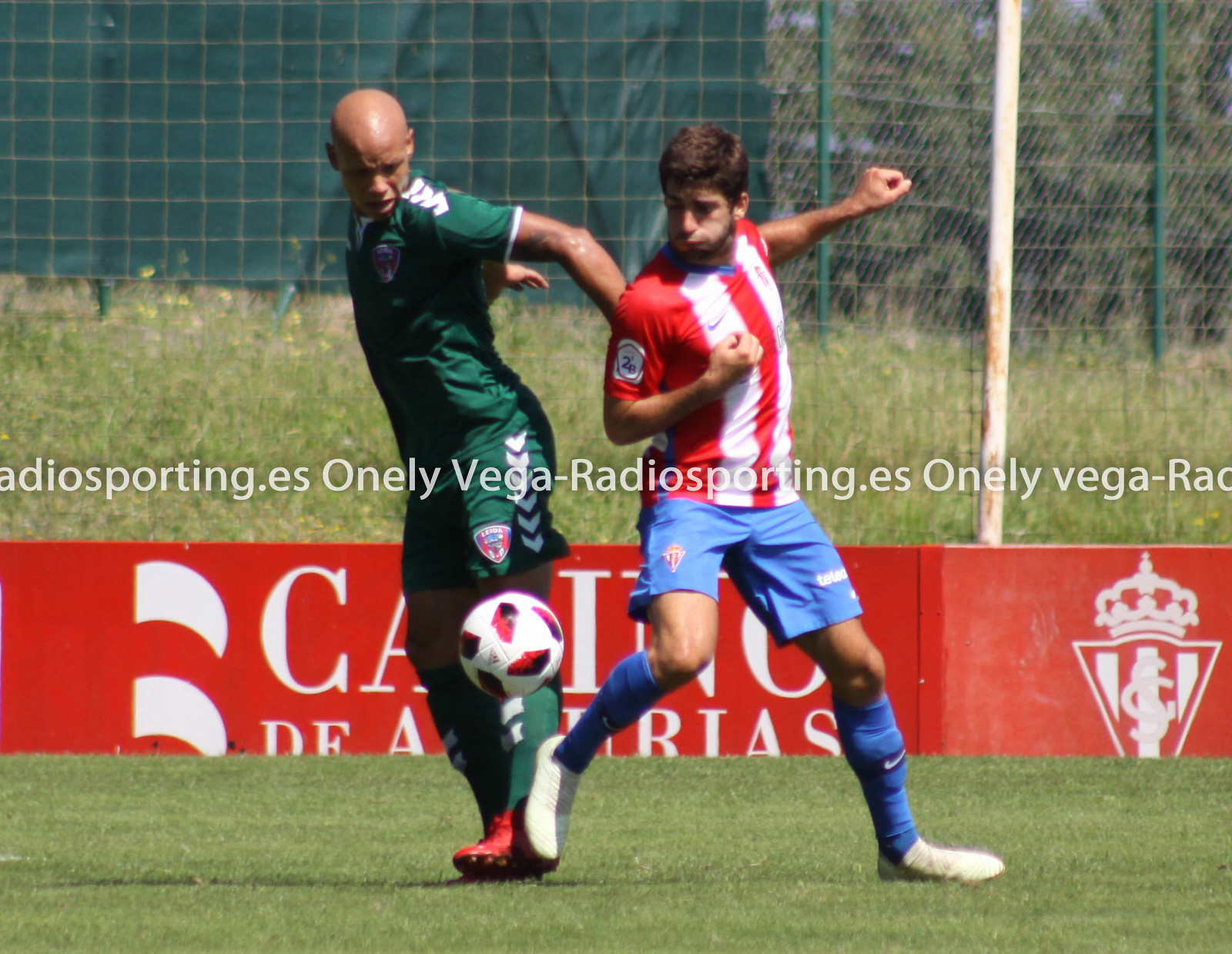In a vibrant soccer match scene, two determined players are captured on a short, well-maintained grass field. Dominating the image is their intense battle for a white and red patterned soccer ball. The player on the left, identifiable by his green jersey adorned with white arrow patterns on the shoulders and sides of the shorts, is bald and intently focused down at the ball. His red cleats contrast sharply with his uniform. Opposing him, the player on the right wears a red jersey with distinctive white stripes, paired with blue shorts and long blue socks, and white cleats. Both players are deeply engaged, their bodies turned in opposite directions, eyes locked on the ball.

In the background, a tall metal wire fence supported by green poles stretches across the scene, partially covered by a green tarp. Closer to the action, a secondary metal wire fence with white poles, now showing signs of rust, stands between the field and the red railings foreground. These red railings are adorned with multiple logos, though many are obscured by the players. Adding a touch of digital branding, the words "onelyvegaradiosporting.es" are repeated in white text across the image, indicating a possible promotional overlay.